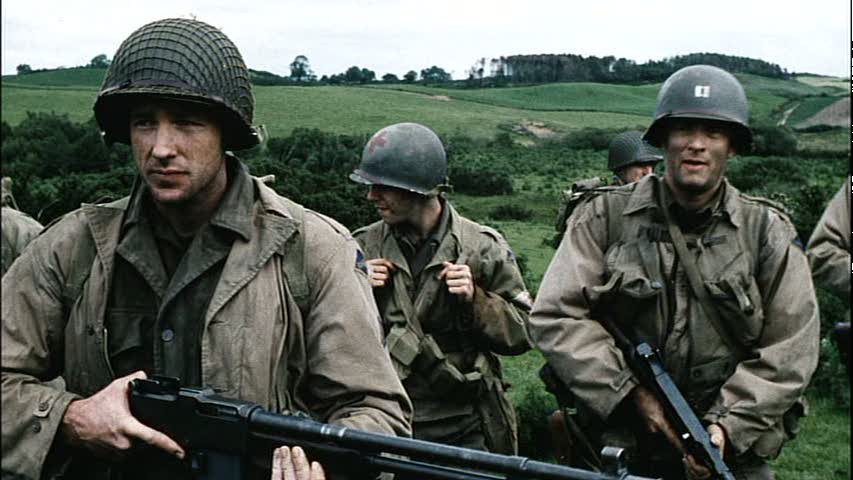In this compelling still from a war-themed TV series or movie, six soldiers are partially visible amidst a grassy, rolling landscape dotted with shrubs and trees. The central figure, who strikingly resembles Tom Hanks, gazes directly at the camera, clad in a traditional army uniform featuring a tan-colored field jacket over a green button-up tunic. His dark green helmet, adorned with netting, sits firmly on his head. To his left, another soldier holds onto a backpack, equipped similarly and looking off to the left. On the far left of the image, a soldier, only partially visible, holds an imposing large automatic machine gun. This weapon, with a black barrel, iron sight at its tip, and a brown woodstock, is showcased prominently. Both soldiers on the far left and far right are mostly cut off at the edges, revealing just an arm or a shoulder. The men appear prepared for action, possibly scouting for the enemy, with their gear suggesting a readiness for combat or reconnaissance.